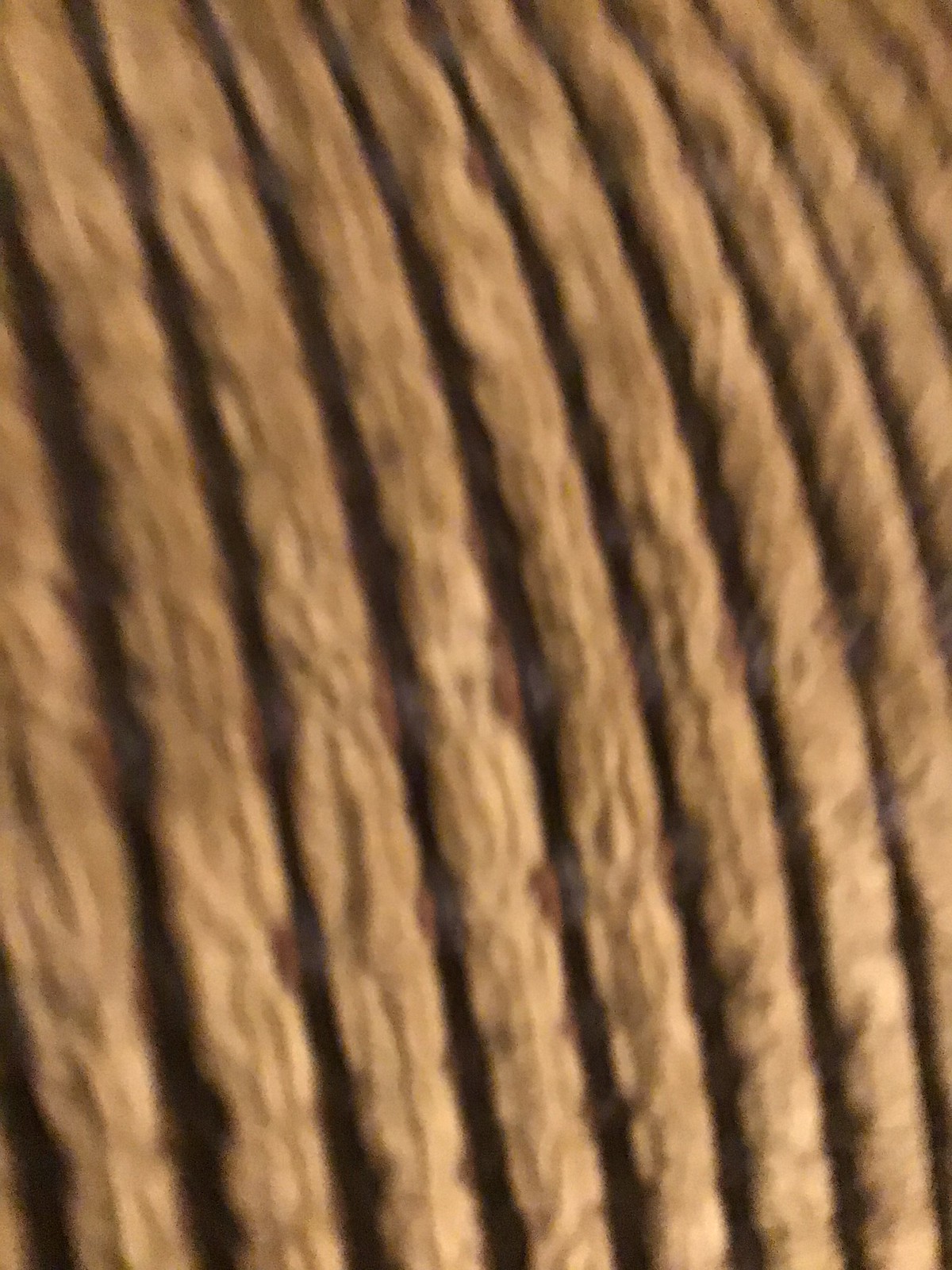The image features a series of long, vertical lines that stretch horizontally across the frame, creating an intriguing visual pattern. The first vertical line measures approximately six inches in length, while the successive lines extend up to about nine inches. Each line is roughly an inch wide and exhibits a light tan color, though they transition into a darker tan at the top before lightening again midway down. These lines are reminiscent of thin ropes, complete with a textured surface that enhances their rope-like appearance. The background is a stark, solid black, which sharply contrasts with the tan lines and accentuates the spacing between each rope-like element.